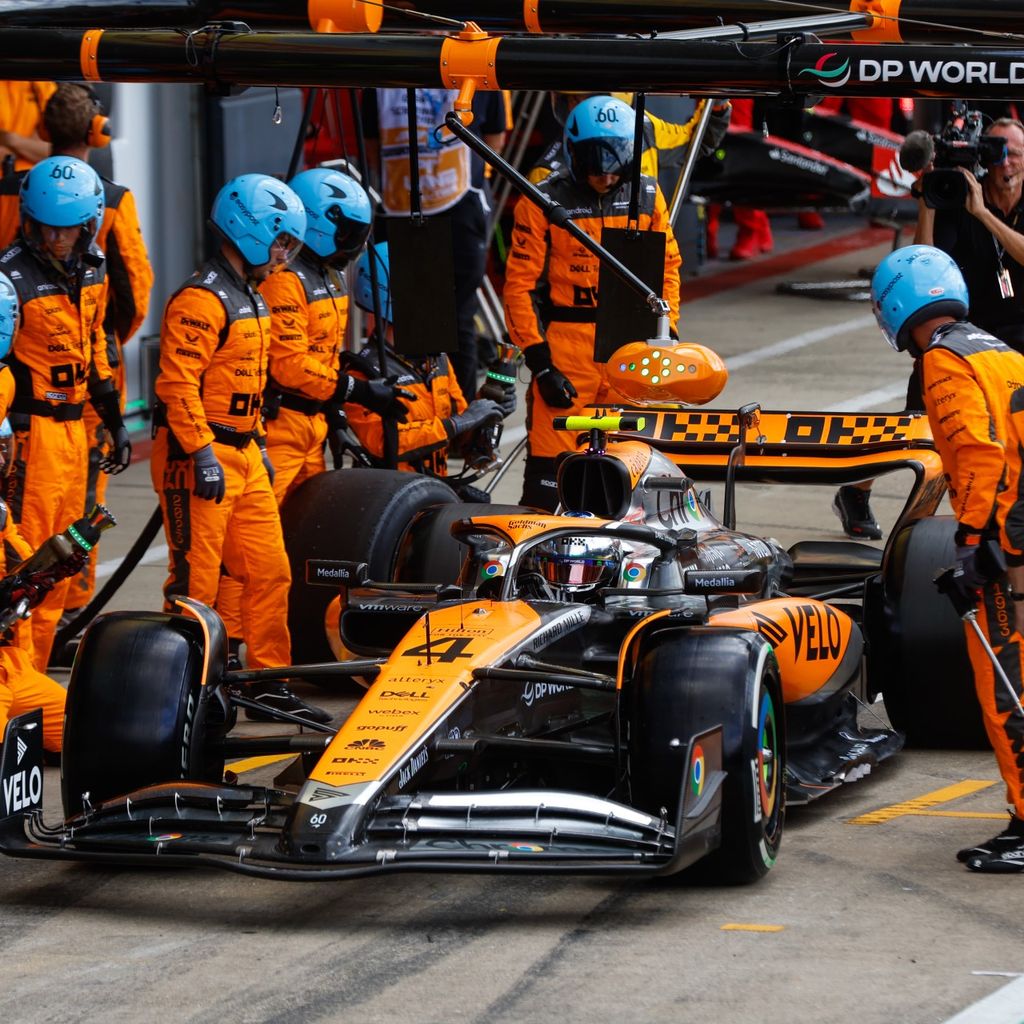In this detailed image, we're presented with a dynamic scene at a pit stop during a high-stakes motor race. An orange Formula 1 race car, prominently featuring the number "4" in black on its front, takes center stage. "VELO" is inscribed on the side of the car, adding to the sleek design elements. The car's branding includes a sign above displaying "DP World" in white letters on a black bar, complemented by a distinctive logo consisting of a red and white swirl with a green stripe stemming from the center.

Surrounding the car is an animated pit crew, all clad in matching orange jumpsuits with black piping and light blue helmets. These helmets feature a logo reminiscent of a boomerang or a playful interpretation of the New England Patriots' helmet symbol. The crew appears focused on their tasks, indicative of a pit stop either just completed or in progress.

In the background, a man in a black shirt is capturing the scene with a camera, adding to the sense of urgency and action. The raceway itself, marked with yellow lines and noticeable skid marks, suggests recent high-speed maneuvers and rapid braking. Additional elements such as large round rubber tires and an implied sense of motion contribute to the overall intensity and realism of the moment depicted.